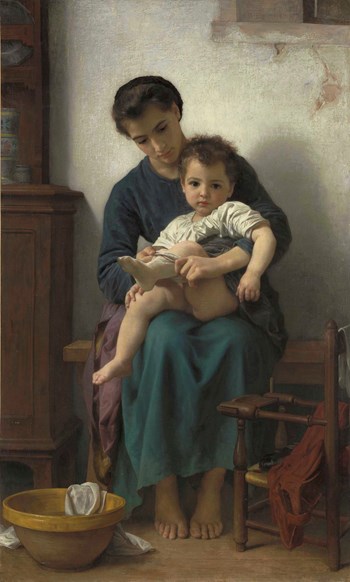This detailed oil painting portrays a realistic scene set indoors in the 19th century. A young woman, possibly a mother, with short brown hair that falls just above her ears, is seated on a wooden bench. She is dressed in a dark green, long-sleeved blouse and an emerald green skirt, and her bare feet rest on the brown floor, revealing all ten toes. In her lap, she tenderly holds a small child with short reddish hair, who is wearing a white shirt and appears to be without a diaper. The child has one sock on, with the mother either putting on or removing the other.

To the right of the woman’s foot, there is a vintage baby seat adorned with a scarf. At her feet is a large yellow bowl containing water and a white cloth. On the left side of the image stands a wooden hutch with a cabinet at the bottom and a shelf on top, adding to the antique ambiance of the room. In the upper part of the painting, a partial view of a window with frames against a cracked white wall provides a touch of natural light.